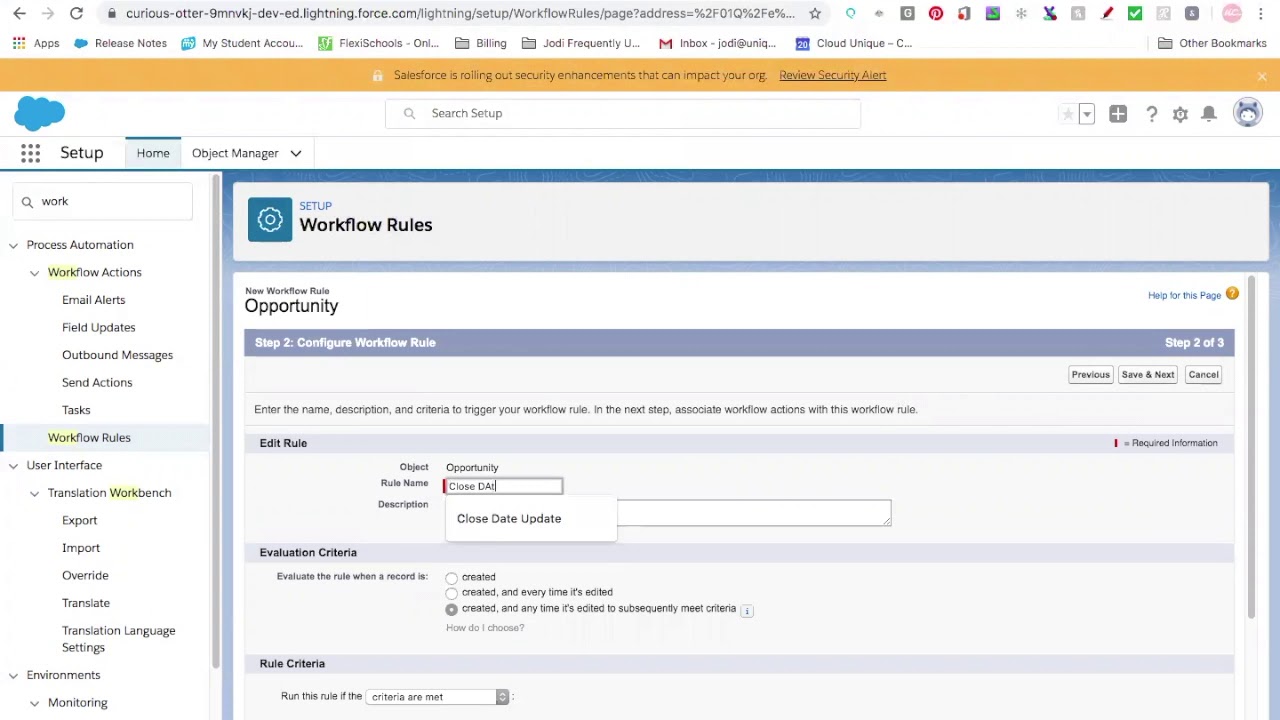The image depicts a detailed page from a workflow rule setup on a website, likely related to a Customer Relationship Management (CRM) tool or similar platform.

At the top of the page, the title "Workflow Rules" is prominently displayed. Directly above, "Setup" is written in blue font above smaller, black text. Below the title, a teal blue box features a circle with rough edges containing text related to an opportunity.

Underneath the teal box, a purple bar indicates the progress of the setup with the text "Step Two: Configure Workflow Rule." This suggests that there were preceding steps and there will be subsequent steps in the process. On the right-hand side, a sidebar outlines various steps with "Step Two" and "Step Three" highlighted, alongside an option to "Edit Rule."

Further details in this section include fields such as "Object: Opportunity," "Rule Name," and "Description" with specific mentions of "Close Date" and "Update." Additionally, it lists "Evaluation Criteria" and "Rule Criteria."

The left-hand side of the page features a navigation panel, starting with a blue illuminated "Setup Home" under which "Object Manager" appears. The search bar located here shows the term "work" has been input. 

Below the search bar, various options are listed such as "Process Auditor," "Window Actions," "Email," "Field," "Outbounds," and "Actions Tasks." The page also includes categories such as "User Interface," "Translation," "Workbench," "Export," "Import," "Override," "Translate," "Transaction," "Language Settings," "Environment," and "Monitoring."

Overall, the page is a detailed part of a sequential setup process for configuring workflow rules, featuring navigation elements, setup instructions, and various criteria and parameters specific to the rule in question.